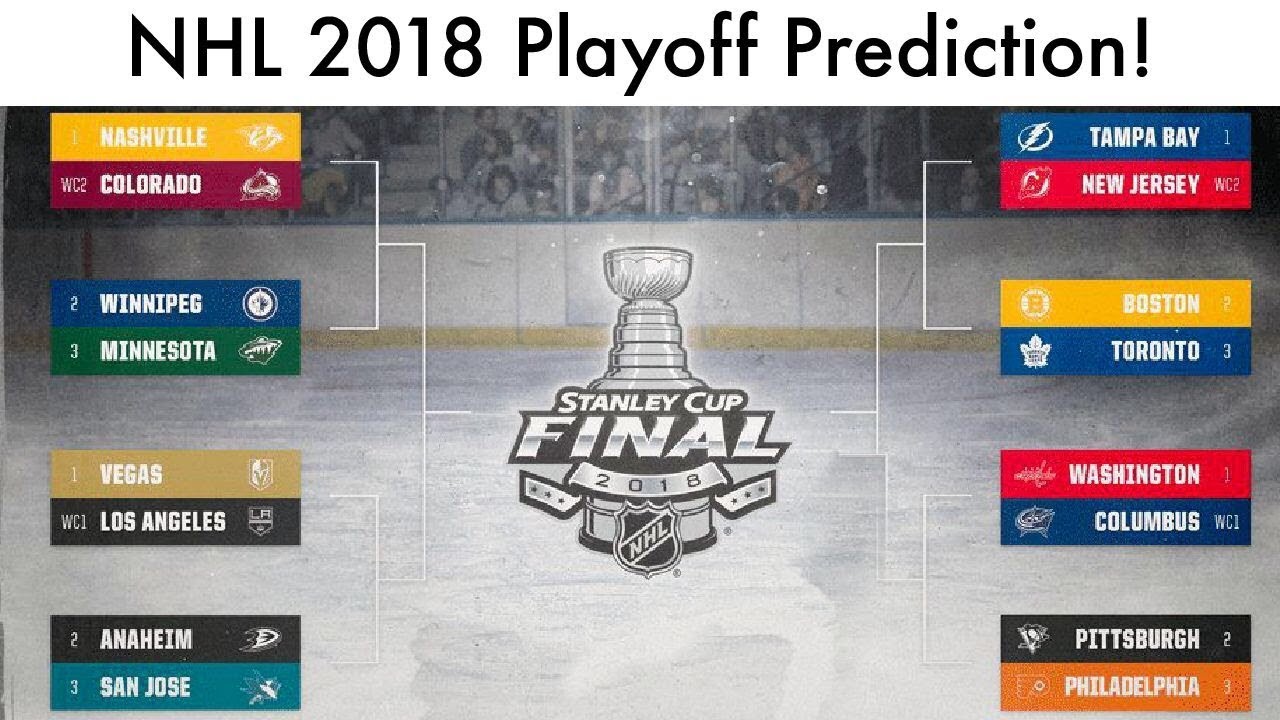This image features an NHL 2018 playoff prediction bracket set against the backdrop of a lively ice skating rink filled with spectators. At the top, the text "NHL 2018 Playoff Prediction" is prominently displayed in black writing on a white background. The centerpiece of the image is a graphic depicting the Stanley Cup trophy, with the words "Stanley Cup Final 2018" beneath it, accompanied by the NHL logo. The bracket showcases the teams participating that year, split into two sides leading to the final matchup. 

On the left side, the matchups are: Nashville vs. Colorado, Winnipeg vs. Minnesota, Vegas vs. Los Angeles, and Anaheim vs. San Jose. On the right side, the matchups are: Tampa Bay vs. New Jersey, Boston vs. Toronto, Washington vs. Columbus, and Pittsburgh vs. Philadelphia. These matchups are displayed in a classic tournament-style bracket, hinting at the progression teams must make towards the Stanley Cup final. The background scenery features a packed NHL stadium, with fans visible behind the glass enclosure surrounding the ice rink, adding to the atmosphere of anticipation and excitement. Despite the detailed layout, there are no specific predictions filled in, making it an open template for fans to speculate on the outcomes.